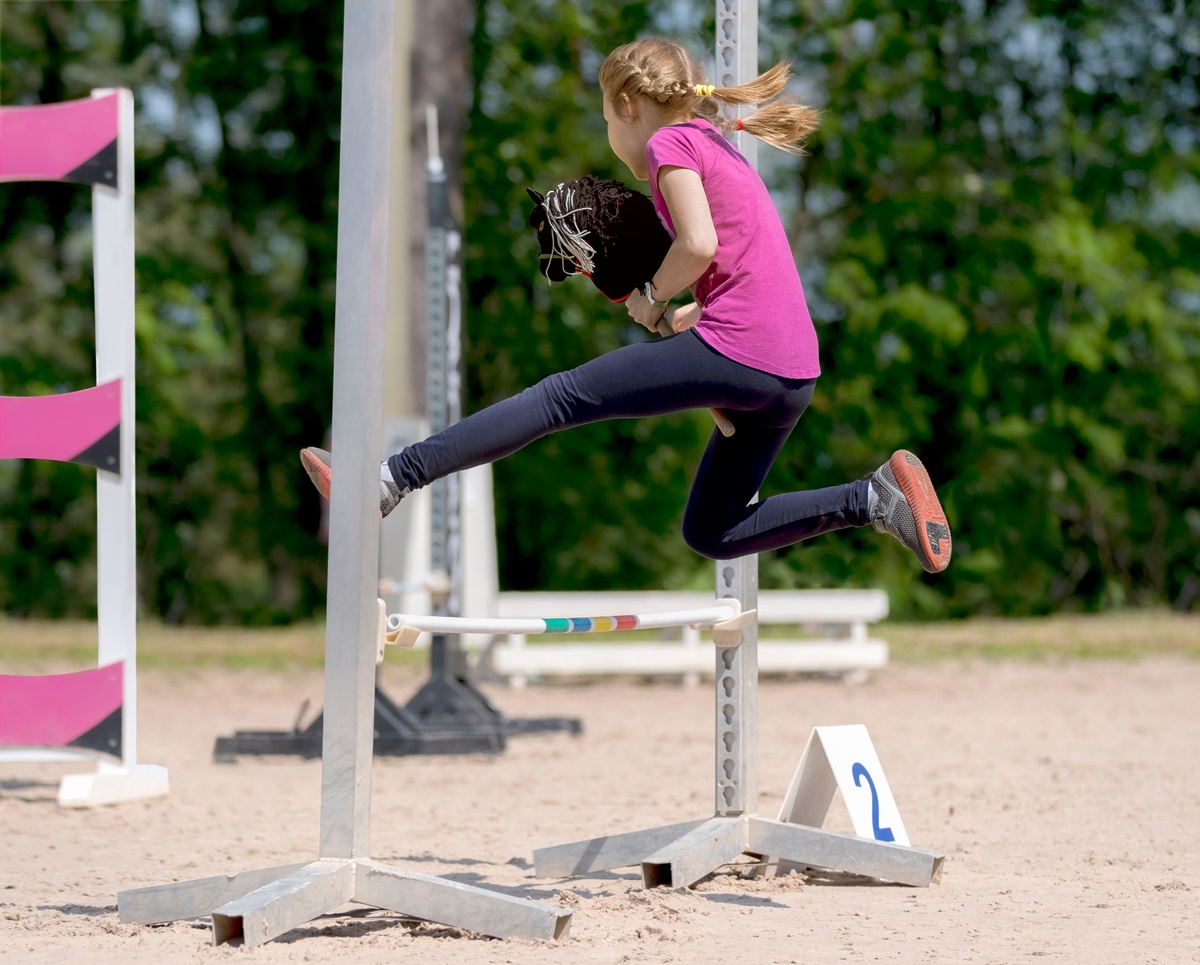In this daytime outdoor photo, a young girl, appearing between seven and nine years old, is captured mid-air as she jumps over an equestrian hurdle at a park-like setting. She has light skin and light brown, braided hair styled into two pigtails. The girl is dressed in dark blue leggings, a dark pink t-shirt, and gray sneakers. She holds a makeshift horse head on a wooden stick, positioned between her legs, simulating the act of riding an imaginary horse. The hurdle she is jumping over has a sign that reads "2" and is approximately one foot off the dirt ground. Behind her, there are additional hurdles, a patch of green grass, and tall trees with glimpses of blue sky poking through.